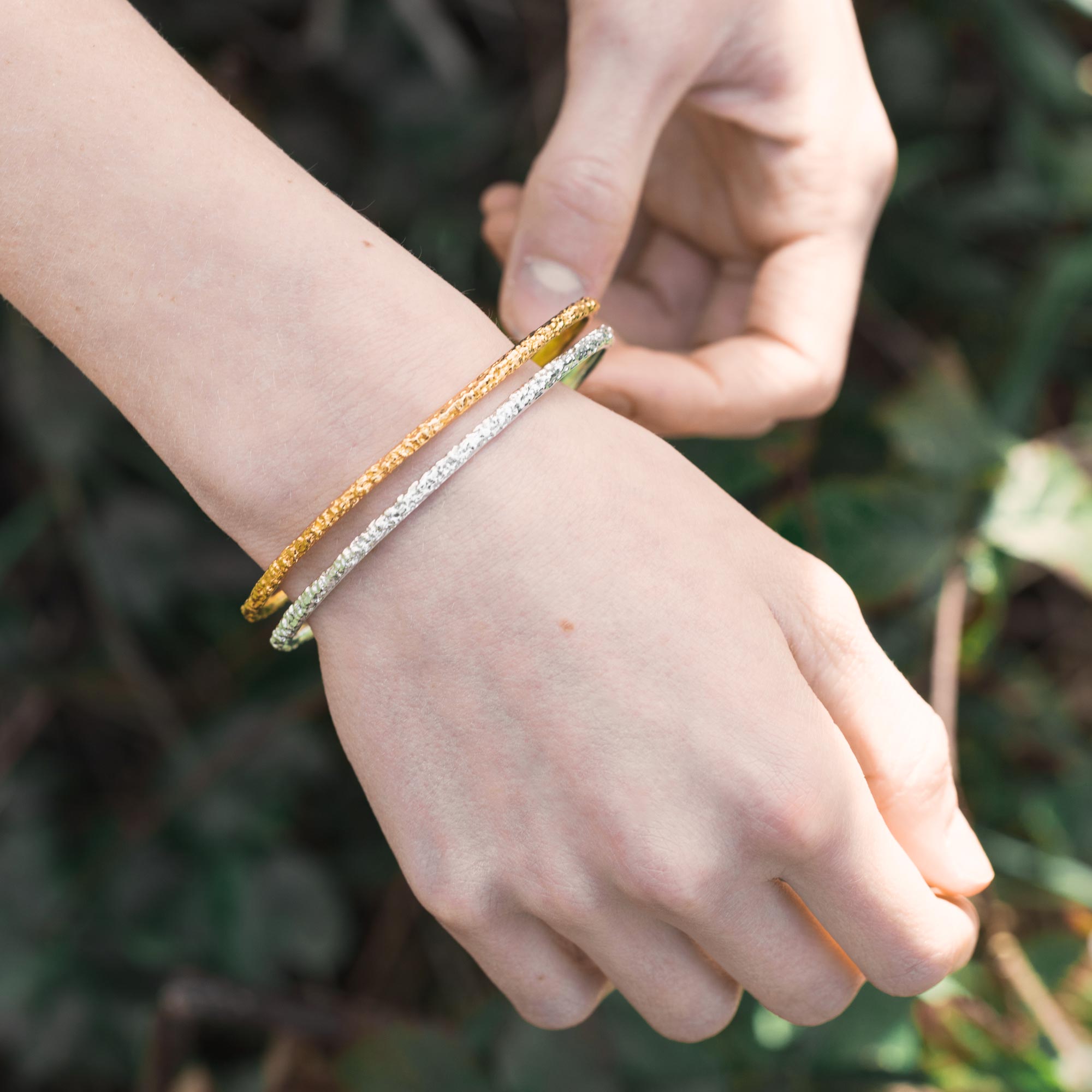This is a full-color, vertically rectangular photograph taken outdoors during the day, utilizing natural lighting. The blurred background consists of out-of-focus greenery, primarily leaves, with a hint of sunlight hitting some foliage in the lower right-hand corner. At the center of the image are two Caucasian hands, which appear delicate and likely belong to a teenage girl, evident from the small size of the wrists and hands. The left hand, emerging from the upper left corner of the frame, is adorned with two bracelets—one silver and the other a gold-copper color—both featuring some detailing. The right hand, coming from the top right, gently holds the bracelets together between the thumb and forefinger. The girl's nails are painted, and a small freckle can be seen on one of her hands.